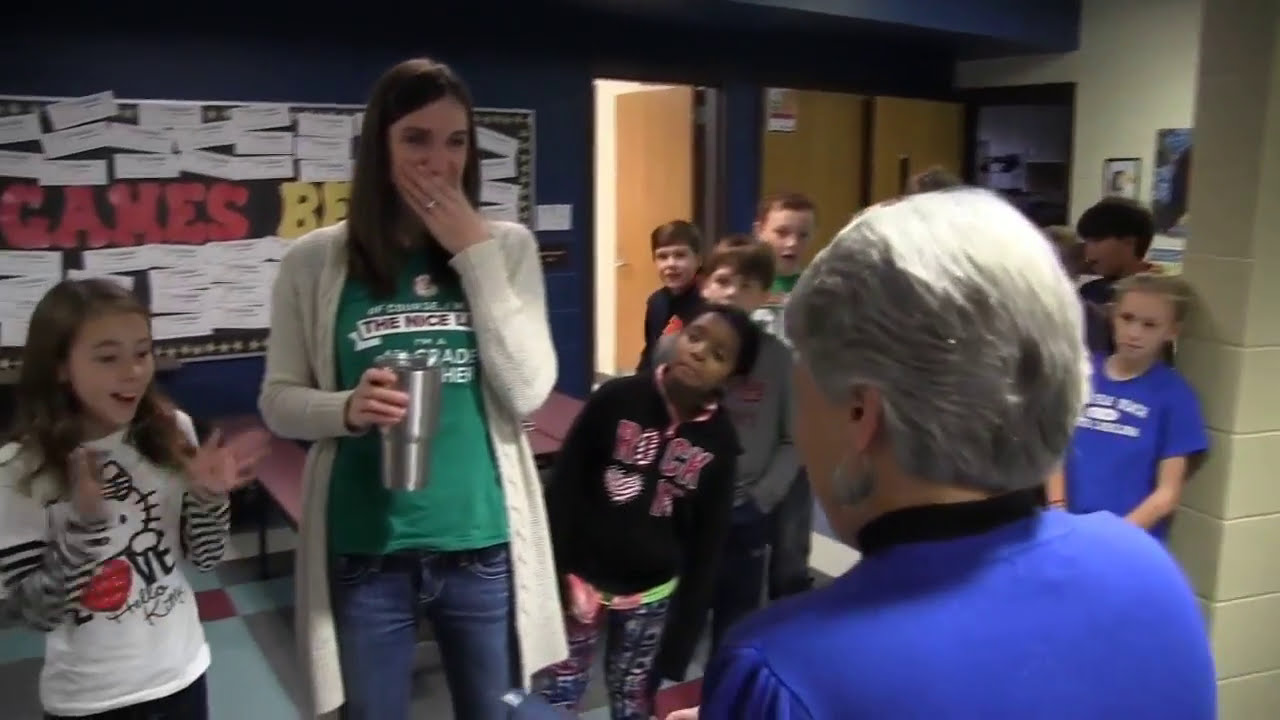The image captures a vibrant scene in a school setting, characterized by a wide rectangular classroom backdrop. The right side features a brick wall and a corner, while the background reveals a navy blue wall adorned with a bulletin board covered in white strips of paper, partially obscured words "games" and "BE" visible. Adjacent are three wooden doors. Dominating the foreground, a woman with dark brown, shoulder-length hair, dressed in a green t-shirt, white sweater, and blue jeans, holds a silver cup in her right hand and covers her mouth with her left, suggesting a smile. To her left stands a younger girl wearing a black and white Hello Kitty shirt, enthusiastically clapping her hands. Many small children cluster in the background, seemingly intrigued. In the image's bottom right corner, another woman, presumed to be older with gray and white short hair, wears a blue shirt and earrings, her back to the camera as she looks onward.